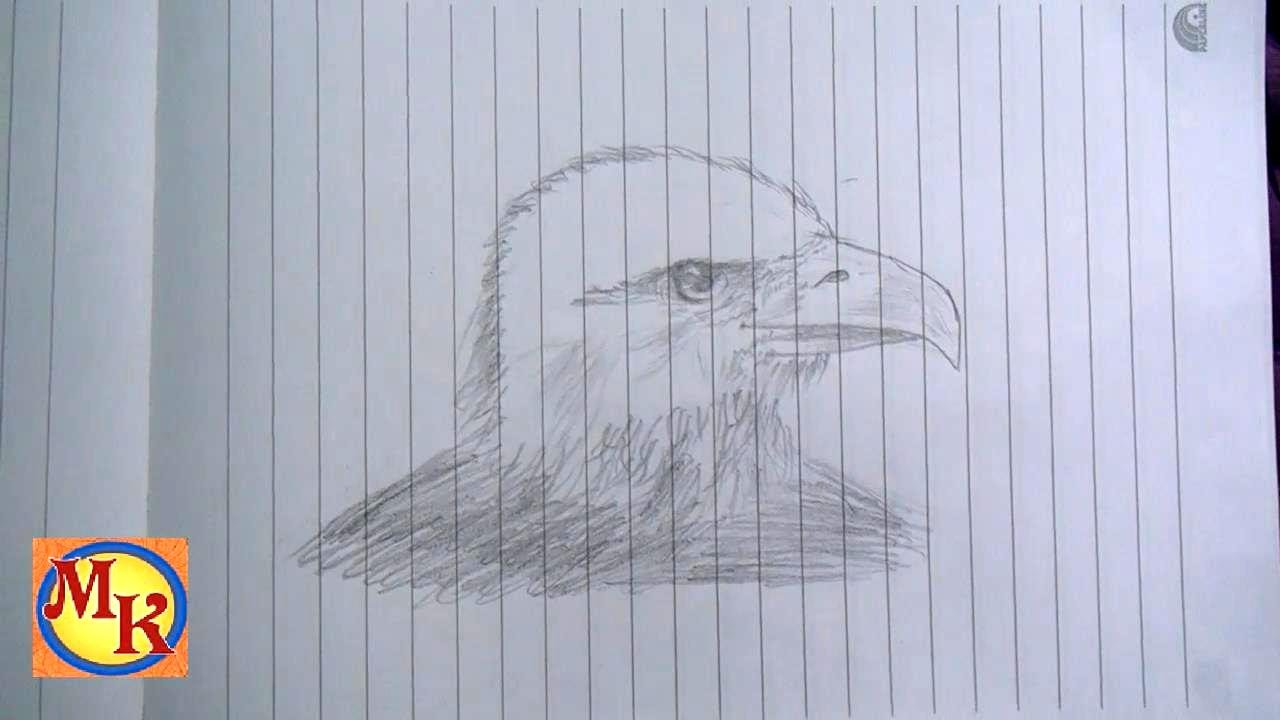This detailed pencil sketch captures the majestic profile of a bald eagle, meticulously drawn on a sheet of lined notebook paper. The paper, oriented vertically, provides a unique backdrop with its gray ruled lines running from top to bottom. The drawing focuses on the right side of the eagle's face and neck, skillfully shaded to reveal intricate details. The eagle's eye is intense and open, showcasing a visible pupil, while the pointed beak features a subtle marking on its side, adding further realism. The artist has expertly conveyed the bird's texture, highlighting fuzziness around the head and neck area.

The sketch occupies the central portion of the page, leaving a margin around its borders. In the lower left-hand corner of the paper, there's a distinct icon: an orange square with a blue circle, which is filled in with yellow and contains large letters "M" and "K" in brown. Additionally, the upper right-hand corner of the sheet features a brand logo, suggesting the origin of the notebook. This beautifully crafted sketch, devoid of any color beyond the gray pencil, effectively captures the noble essence of the bald eagle against an everyday backdrop.